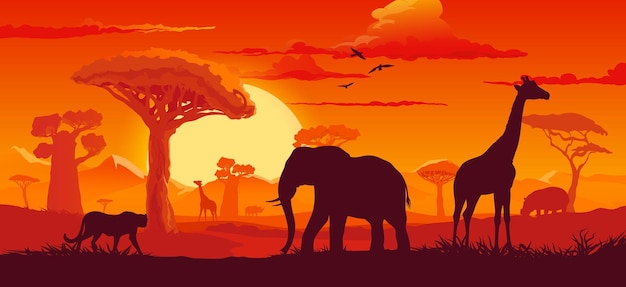This image presents a digitally created African safari scene predominantly in black silhouettes contrasting against a vibrant orange-red sky. In the foreground, three distinctive black silhouettes stand on a grassy area: a cheetah on the left, an elephant in the center, and a giraffe on the right. This layer of ground is depicted in black, providing a stark contrast to the colorful background. Further behind, the landscape continues in a reddish hue, showcasing more silhouettes of African trees and another giraffe. Additionally, a hippopotamus silhouette is visible deeper in the backdrop. The sky is an exquisite display of warm tones, featuring a large sun peeking out from the left side, partially obscured by orange silhouettes of trees. The sky is dotted with three black birds in flight, complementing the rich orange canvas, while red clouds drift overhead.